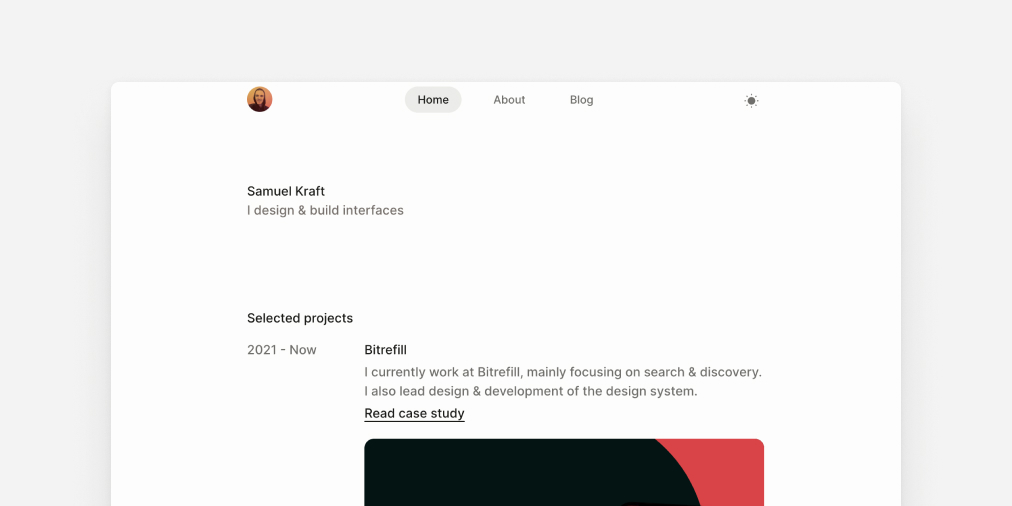This image depicts a blog webpage belonging to Samuel Kraft, a designer specializing in interface design and development. In the top left corner, a digital photo of Samuel Kraft is displayed. The webpage features navigation categories including "Home," "About," and "Blog." Samuel Kraft introduces himself with the statement: "I design and build interfaces." Highlighting his professional experience, the page specifies his work on selected projects from 2021 onwards, primarily at Bitrofio, where he focuses on search and discovery. Additionally, he leads the design and development of the company's design system, with a case study provided. The color palette of the page includes black and red text against a white background, with no other notable details present.